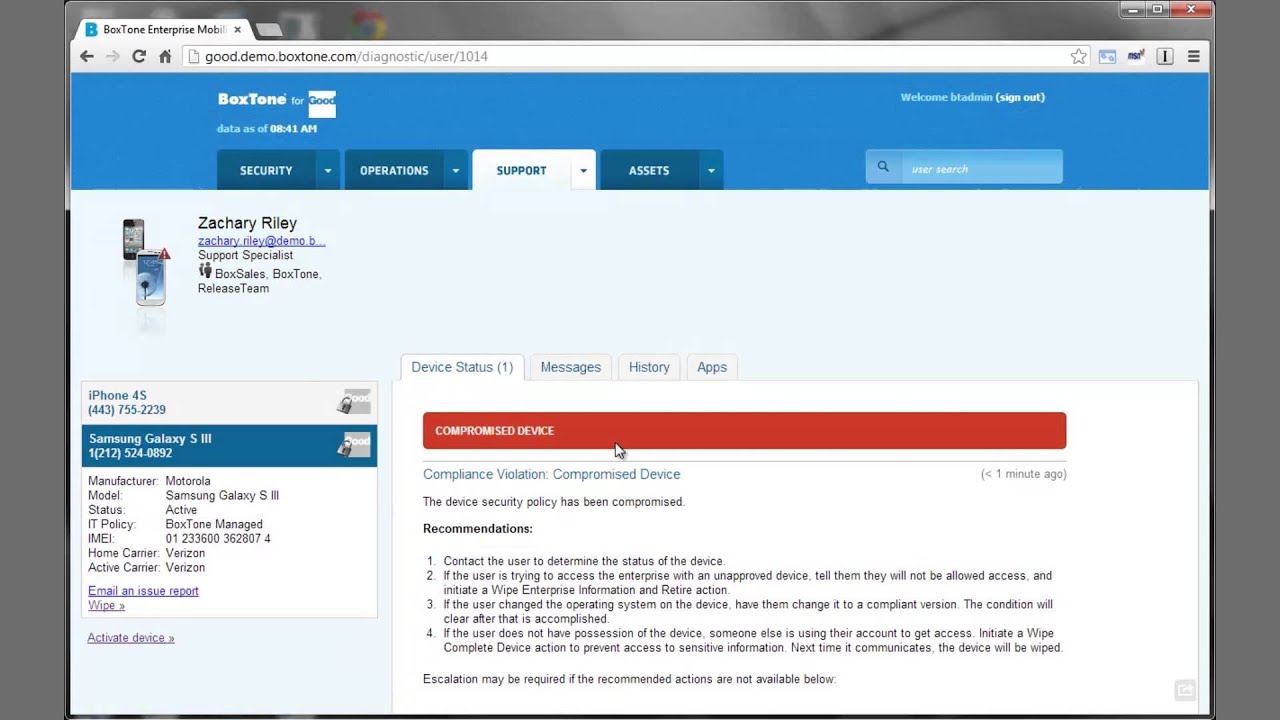**Detailed Caption:**

The screenshot displays a desktop web page providing detailed diagnostic information about a cell phone, hosted on the Boxtone Enterprise Mobile platform. At the top of the browser tab, the website is labeled "Boxtone Enterprise Mobile," though the full label is cut off. The URL reads "good.demo.boxtone.com/diagnostic/user/1014."

At the very top of the web page, there is a blue header. On the left, it reads "Boxtone for good" with data timestamped at "8:41 AM". On the right side of the header, the page greets the logged-in user with "Welcome BT admin" followed by a "Sign Out" option in parentheses.

Below the header are several navigational tabs: 
1. "Security" (dark blue)
2. "Operations" (dark blue)
3. "Support" (white, selected tab)
4. "Assets" (dark blue)
Additionally, to the far right, there is a user search bar labeled "User Search."

Further down, the main content of the page begins with user details: "Zachary Riley." His email is partially shown in blue as "zachary.riley@demo.b...", followed by his role "Support Specialist," and team affiliations, "Box Sales" and "Boxtone Release Team." To the left of this information, there is an image of two smartphones.

The core of the page details smartphone information in a white box. At the top, it lists an iPhone 4S, identified by the number "443-755-2239" with a "good" status indicated in a light gray box accompanied by a lock icon. Below this entry, there is another detailed entry for a Samsung Galaxy S3 (number: "1-212-524-0892" featuring a similar "good" logo).

The box then lists specific details for the Samsung Galaxy S3:
- Manufacturer: Motorola
- Model: Samsung Galaxy S3
- Status: Active
- IT Policy: Boxtone Managed
- IMEI: 012336003628074
- Home Carrier: Verizon
- Active Carrier: Verizon
- Email: Email and Issue Report (in blue)
- Action: Wipe

Lastly, beneath the white information box, there is an "Activate Device" button.